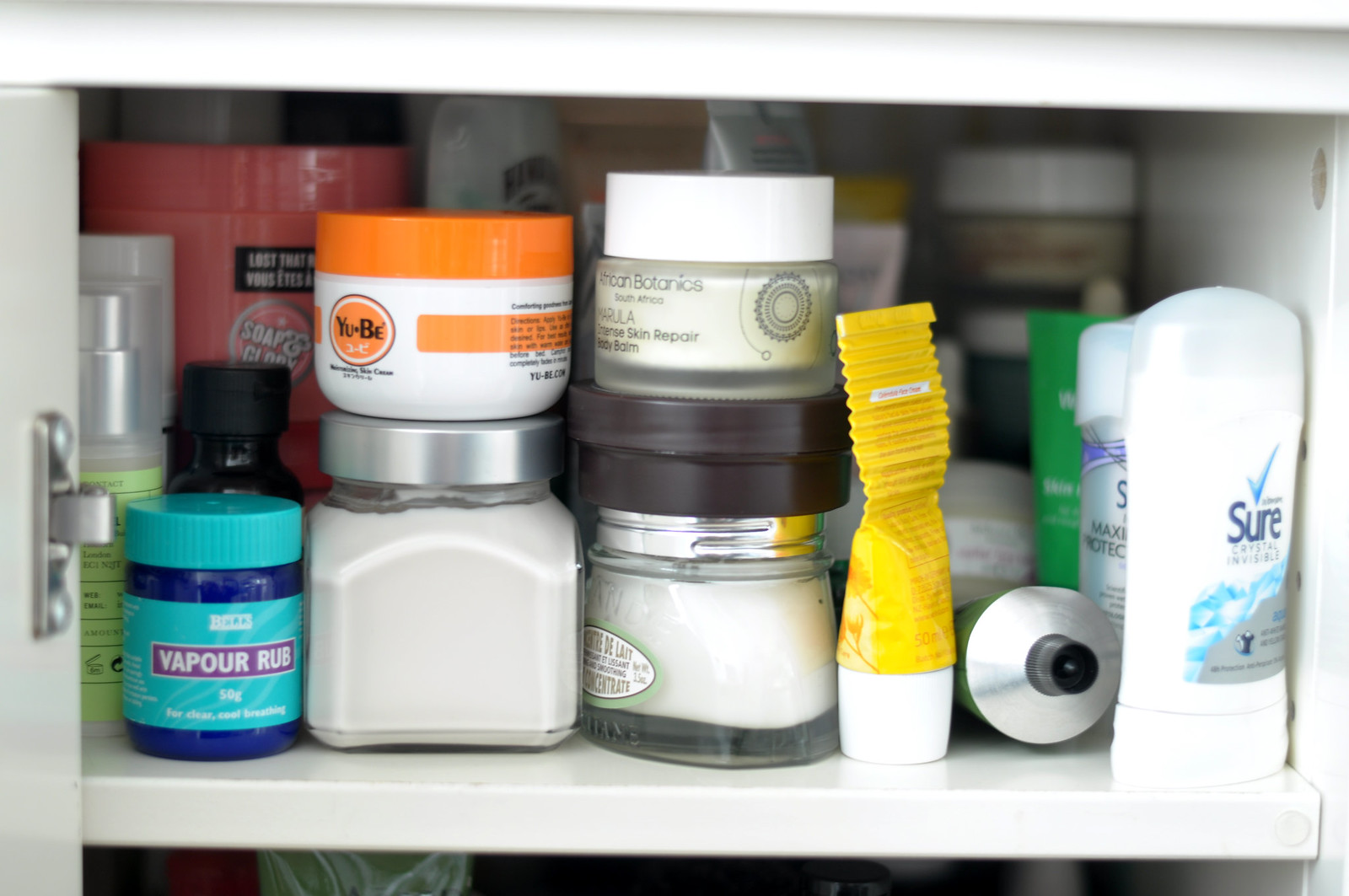The photograph showcases an array of medicinal products neatly organized inside a white wooden cabinet. From left to right, the lineup begins with a blue bottle of vapor rub, distinguished by its light blue paper seal and matching blue lid. Adjacent to it, a large clear glass jar contains an unidentified powder, topped with a small white tube featuring a yellow-orange lid—presumably some kind of lotion. Following these, two more glass vials hold other powders, their labels unreadable. Next in line is a partially used yellow toothpaste tube capped with a white lid. The scene also includes two types of women's deodorant labeled "Sure," both housed in white cases. Beyond these primary items, a variety of other products are partially visible but remain out of focus and obscured. The cabinet's clean, white wooden interior provides a neutral backdrop that highlights the variety of stored items.